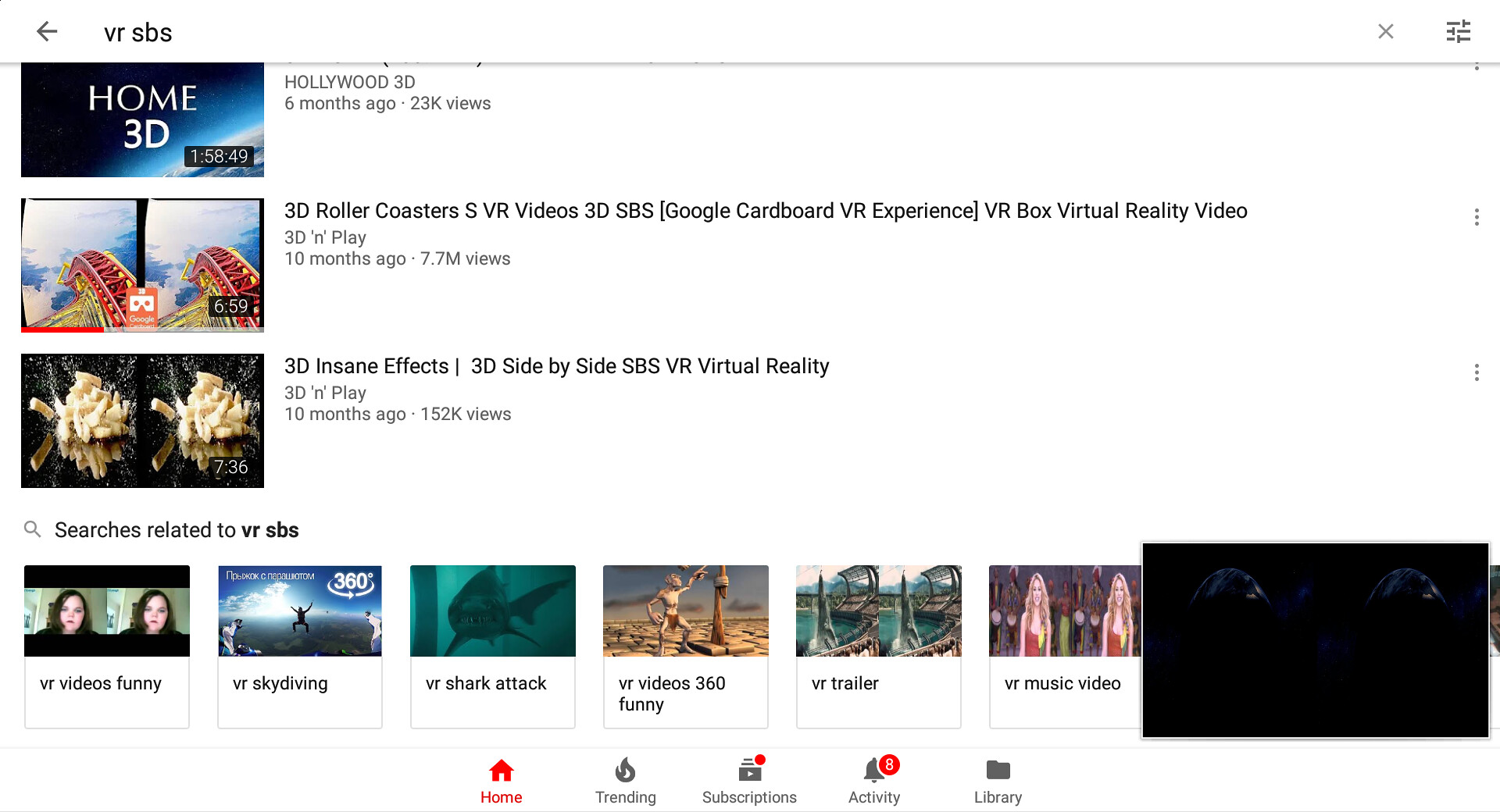A detailed photo of a computer screen displays a search engine results page for the query "VR SBS". In the search bar, the term "VR SBS" is clearly visible. Below the search bar, the first search result features a thumbnail image of a rectangular shape and labels "Home 3D" alongside "Hollywood 3D." This listing shows it was posted six months ago and has garnered 23K views.

The subsequent result showcases a thumbnail with two side-by-side roller coaster images. The title next to it reads, "3D Roller Coasters SVR Videos 3D SBS Google Cardboard VR Experience VR Box for Virtual Reality Video," clearly optimized with multiple keywords. 

Following this is another thumbnail depicting what appears to be french fries, again duplicated side-by-side. The accompanying title is "3D Insane Effects 3D Side-by-Side SBS VR Virtual Reality."

Further down the page, under the heading "Searches related to VR SBS," several additional thumbnails appear. These include, from left to right, "VR Videos Funny," "VR Skydiving," "VR Shark Attack," "VR Videos 360," "Funny VR Trailer," and "VR Music Video."

In the bottom right corner of the screen, a small black rectangle appears, resembling a picture-in-picture element, containing a blue half-circle.

Lastly, the bottom navigation bar of the screen displays various icons for "Home," "Trending," "Subscriptions," "Activity," and "Library."